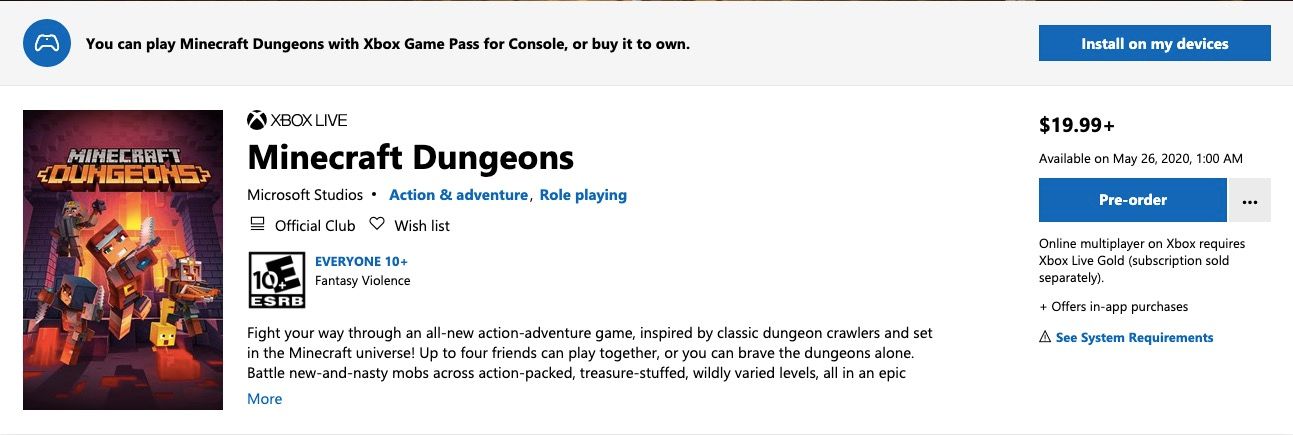A detailed pop-up window from a computer screen advertises "Minecraft Dungeons." At the top, there's a gray bar featuring a small blue circle with a white game controller icon. Beside this icon, black text reads, "You can play Minecraft Dungeons with Xbox Game Pass for console or buy it to own." Below, a prominent blue button labeled "Install on my device" is displayed. The game's colorful cover art is shown, resembling a LEGO-inspired design, with "Minecraft Dungeons" prominently displayed in black text. An "Xbox Live" icon appears next to the game's title. Further details describe the game as part of the "Microsoft Studios" collection, categorized under "Action and Adventure Role Playing" in blue text.

Additional information includes an "Official Club Wishlist" option and an ESRB rating of "E10+ Everyone 10 and up" for fantasy violence. A brief description highlights the game's features: "Fight your way through an all-new action-adventure game inspired by classic dungeon crawlers and set in the Minecraft universe. Up to four friends can play together, or you can tackle the dungeons alone. Battle new and nasty mobs across action-packed, treasure-stuffed, wildly varied fields, all in an epic..." with an invitation to "click more" to read further.

The game is priced at $19.99 and was made available on May 26th, 2020, at 1 am. Pre-orders can be made by pressing the blue button, catering to dedicated gamers and fans of the Minecraft franchise.